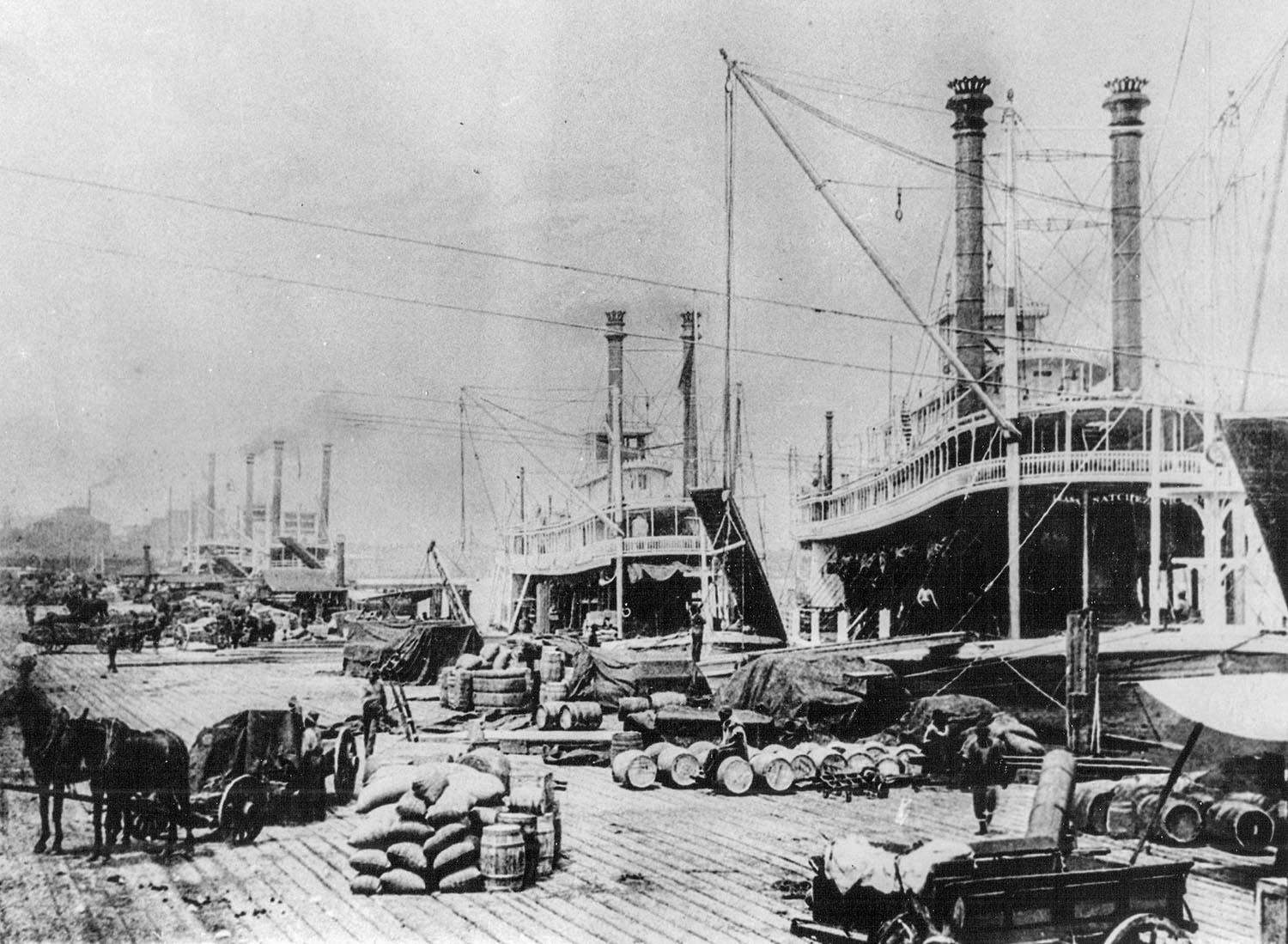This vintage black-and-white photograph captures a bustling harbor scene, likely from the 1920s or 30s. On a clear, cloudless day, the wooden pier is crowded with activity. Along the right-hand side of the dock, three large steamboats, all featuring two-tiered designs with twin smokestacks, are docked. Steam billows from their stacks, and an intricate web of ropes is visible, both atop and dangling from the boats. The busy pier is populated with workers, horses, and carts. Two horses are hitched to a cart on the left side, while other wagons stand independently. Barrels and sacks, neatly stacked in rows, are scattered across the pier, adding to the industrious atmosphere as the people move about, tending to the various cargo and tasks.